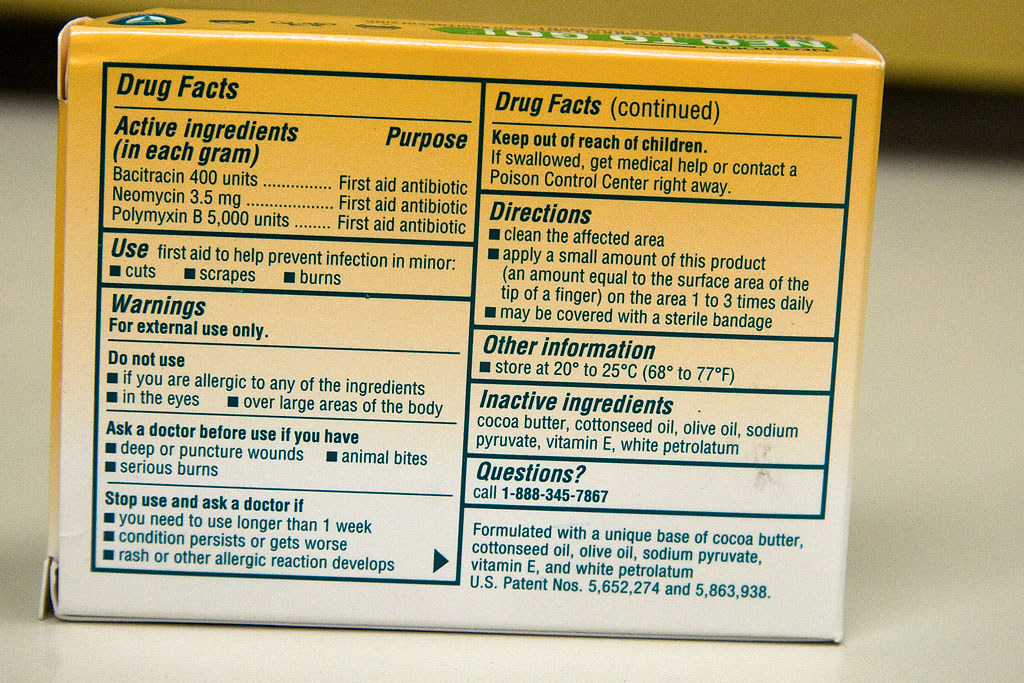In the image, the ground is blanketed in white, transitioning to a yellow sky above, with a distinct black stripe separating the two. Centrally placed is a box featuring a prominent green label at the top which reads "NEO2GO." The back of the box displays detailed drug facts.

The label specifies that the active ingredients per gram are: Vasodilatan with 400 units, First Aid Antibiotic Bacitracin with 3.5 milligrams, and First Aid Antibiotic Polymyxin B with 5,000 units. 

In the top right corner, additional drug facts are outlined, including key factors such as usage for children as a medical aid and the importance of immediate contact with a control center for urgent situations. The product is indicated for first aid to prevent infections in minor cuts, scrapes, and burns. Directions advise applying a small amount, equivalent to the surface area of the tip of a finger, to the affected area. 

Storage recommendations are between 20ºC and 25ºC. The inactive ingredients listed include cocoa butter, cottonseed oil, and olive oil. For any questions, consumers are advised to call 1-888-345-7877.

Additionally, the box advises discontinuing use if symptoms persist for more than one week or if allergic reactions such as rash occur. It highlights the necessity of consulting a healthcare provider before using on deep puncture wounds, animal bites, serious burns, or if used on large areas of the body. The formulation is noted for its unique base of cocoa butter, cottonseed oil, olive oil, sodium pyruvate, vitamin E, and microcrystalline substances.